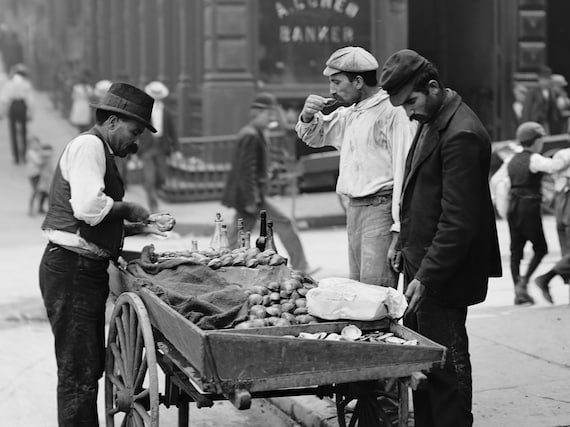In this black and white photograph, likely from the late 1800s to early 1900s, a scene unfolds on a bustling city street, possibly in a coastal town. At the center, a wooden cart, reminiscent of a wheelbarrow with two large wooden wheels, is piled high with oysters. The vendor, positioned to the left of the cart, wears a dark vest over a long-sleeved white shirt with the sleeves rolled up, and a little fedora atop his head. His bushy mustache matches the era's style. He is in the midst of shucking an oyster, holding it in one hand while his other hand manages a bottle of vinegar set on the cart. To the right of the cart, two men in working-class clothes inspect the goods. The man closest to the cart is dressed in a dark jacket and pants, with a dark hat, and reaches toward the cart, perhaps selecting an oyster. Next to him, another man in a light-colored shirt and hat, appearing to be sampling an oyster. His shirt, notably dirtied, suggests the toils of the era. 

The street itself is vibrant with activity. In the background, various figures move about—a few little kids across the street, more pedestrians shuffling past buildings, adding life to this historic moment. A prominent signage for a bank is visible slightly off-center, grounding the photograph with a sense of place. The concrete road beneath and the sidewalk beside it frame this candid glimpse into a past daily life, retaining a timeless aura through its monochrome presentation.